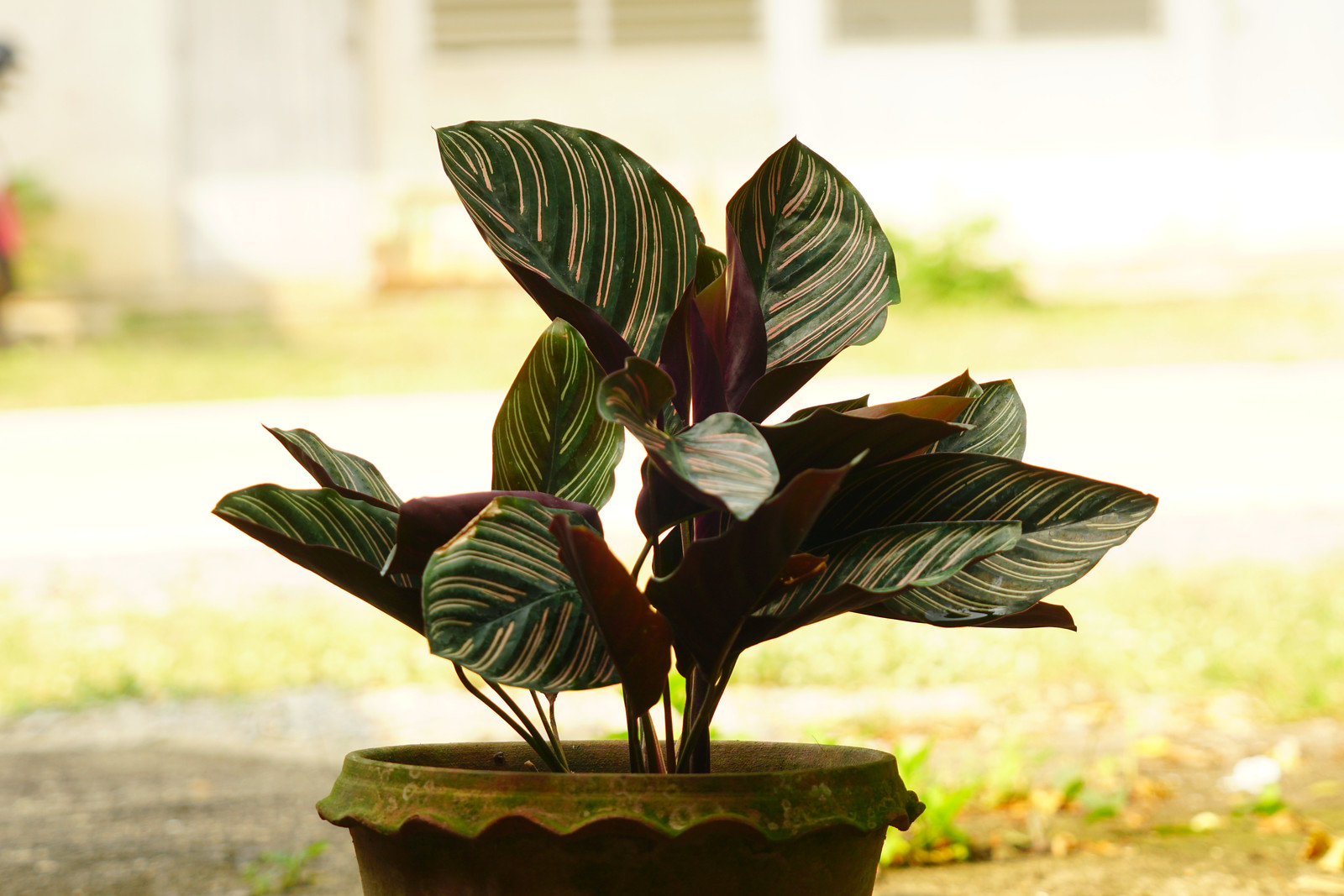In a bright outdoor setting, the image centers on a potted plant situated in the foreground. The pot is predominantly brown with a wavy artistic design around the lip, incorporating an array of red, green, and brown hues. The plant within the pot features large leaves, primarily green with striking yellow and light brown stripes. The undersides of the leaves display a maroon-red tint, enhancing their vibrant appearance. Beyond the potted plant, the yard transitions into a sidewalk before returning to more grassy areas. In the upper third of the image, two white garage doors are centered, providing a backdrop and anchoring the scene in a sunlit outdoor space.